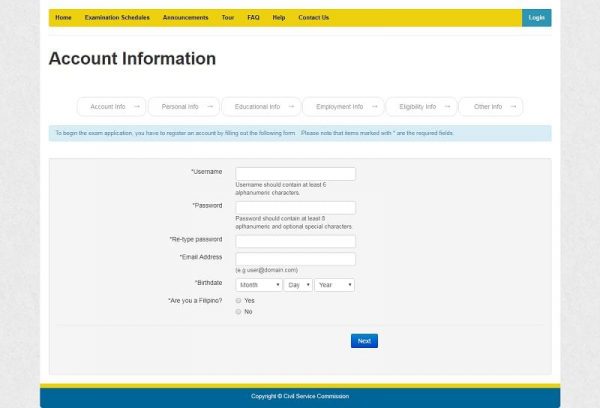The web page is titled "Account Information," prominently displayed in large, bold, black text. A yellow navigation bar spans the top of the page, featuring menu items such as Home, Examination Schedules, Announcements, Tour, FAQ, Help, and Contact Us, all written in black text. To the far right of this yellow bar is a small, blue box containing the white text "Log In."

Just below the navigation bar, the page features a thin yellow line followed by a thick blue bar. This blue bar displays the text "Copyright Something Service Commission" in white. 

The main content area of the page is predominantly white with light gray accents. It hosts a menu with the following categories: Account Info, Personal Info, Educational Info, Employment Info, Eligibility Info, and Other Info. 

Several form fields are arranged below these headings, ready for user input. These fields include Username, Password, Retype Password, Email Address, Birth Date, and a question "Are You a Filipino?" Near the bottom of this section is a blue box containing the word "Next," indicating the next step in the process.